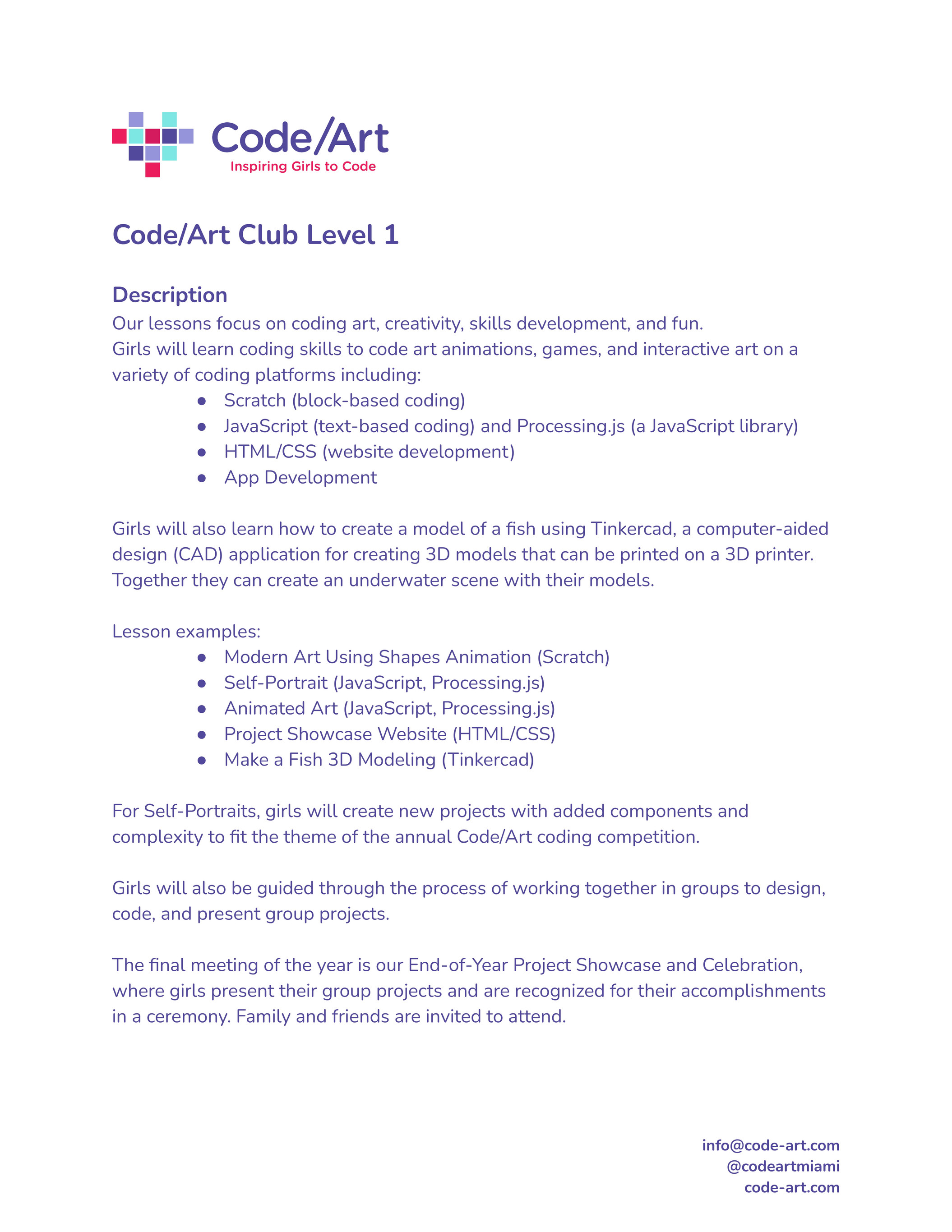The image is a detailed informational page with a white background and light purplish-blue text. At the top, a blue, red, and purple heart logo sits next to the title "Code/Art: Inspiring Girls to Code." This page describes the Code/Art Club Level One with a focus on coding, art, creativity, skills development, and fun. The lessons teach girls coding skills for creating art animations, games, and interactive art on various platforms, such as Scratch (block-based coding), JavaScript (text-based coding), Processing.js (a JavaScript library), HTML/CSS for website development, and app development.

Additionally, girls will learn to create a 3D model of a fish using Tinkercad, a computer-aided design (CAD) application, which can be printed on a 3D printer. Together, they will complete an underwater scene featuring their 3D models.

The page includes lesson examples such as modern art using shapes, Scratch animations, self-portraits using JavaScript with Processing.js, animated art with Processing.js, creating project showcase websites using HTML/CSS, and making a 3D fish using Tinkercad.

For the self-portrait projects, girls will add new components and complexity to align with the theme of the annual Code/Art Coding Competition. They will also work in groups to design, code, and present collaborative projects. The final meeting of the year will feature an end-of-year project showcase and celebration where girls present their group projects and are recognized for their achievements. Family and friends are invited to this ceremony. Contact information is provided at the bottom right: info@code-art.com, @codeartmiami, and code-art.com.